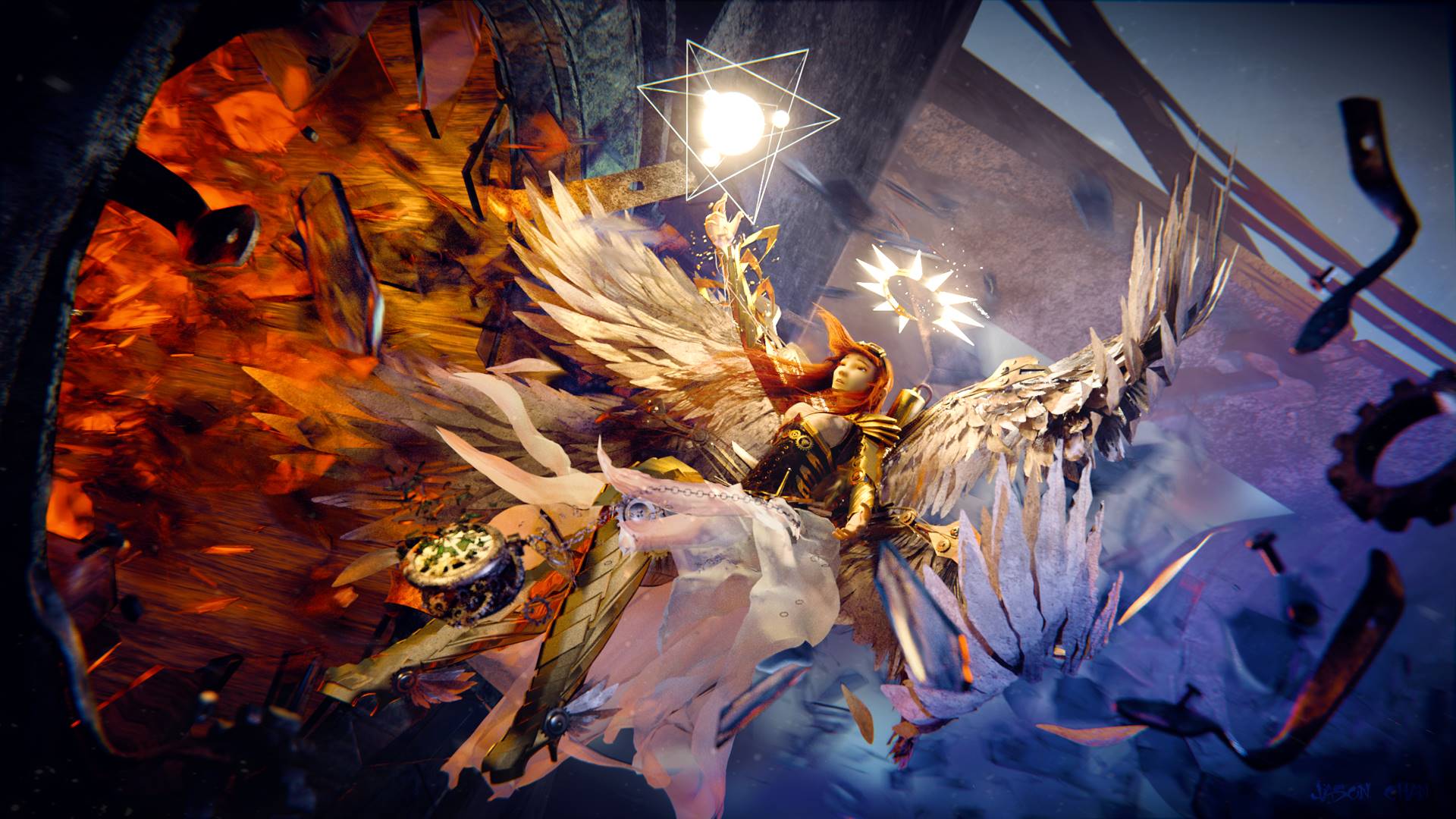The image features a computer-animated, photorealistic fantasy scene dominated by an angelic female figure with striking orange hair and large, feathery white wings. The woman, clad in a detailed white dress with a breastplate and gold shin guards, is depicted floating or falling backward through a vibrant and dynamic sky, her right arm outstretched as if in need of assistance. The background is a blend of fiery reds and dark oranges to the left, evoking the sense of an explosion or a cauldron of flames, while the right side transitions into serene blues. Next to the woman, a geometric pyramid, seemingly composed of translucent layers and emitting bright light, adds an element of mysticism. Additionally, a glowing sunflower-like flower hovers to the right of her. The overall composition is a cacophony of color and form, capturing a moment of dramatic, surreal beauty in what appears to be a celestial or fantastical setting.